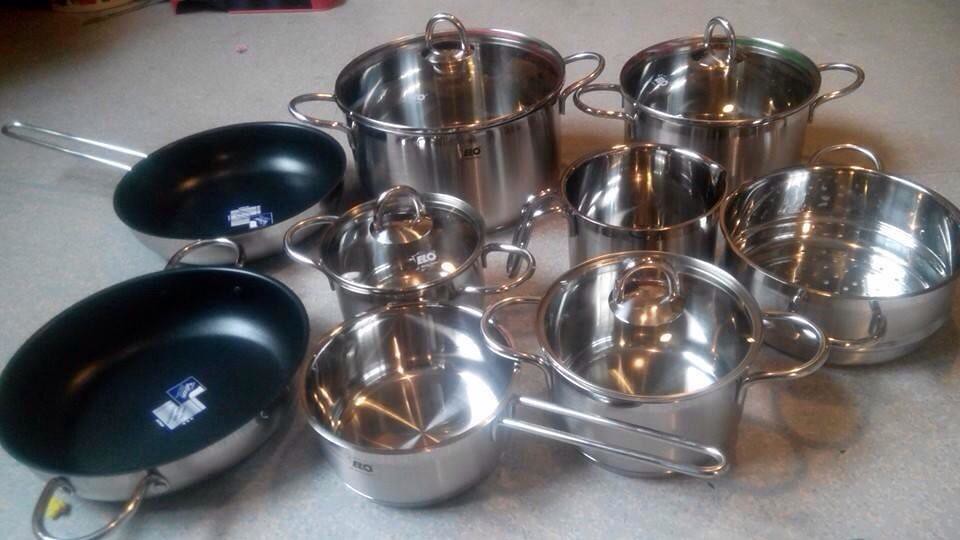This image features an extensive, brand-new set of stainless steel cookware with a brushed silver finish, meticulously arranged on a faint marble-patterned white background. The collection includes nine vessels, each with clear lids that have central circular metallic handles. There are four stock pots of varying sizes: two larger ones in the back, ideal for soup or stew, and two smaller ones in the foreground, all equipped with looped handles on either side. The set also contains two saucepans—one larger with double handles and one smaller with a single long handle, both without lids. Additionally, there is a colander or steamer insert, designed to fit into one of the other pots. Completing the set are two skillets—one resembling a wok with higher edges and a pair of side handles, and another with a long handle. Both skillets feature a black nonstick interior coating and have blue and white labels, indicating they are part of the brand-new set.